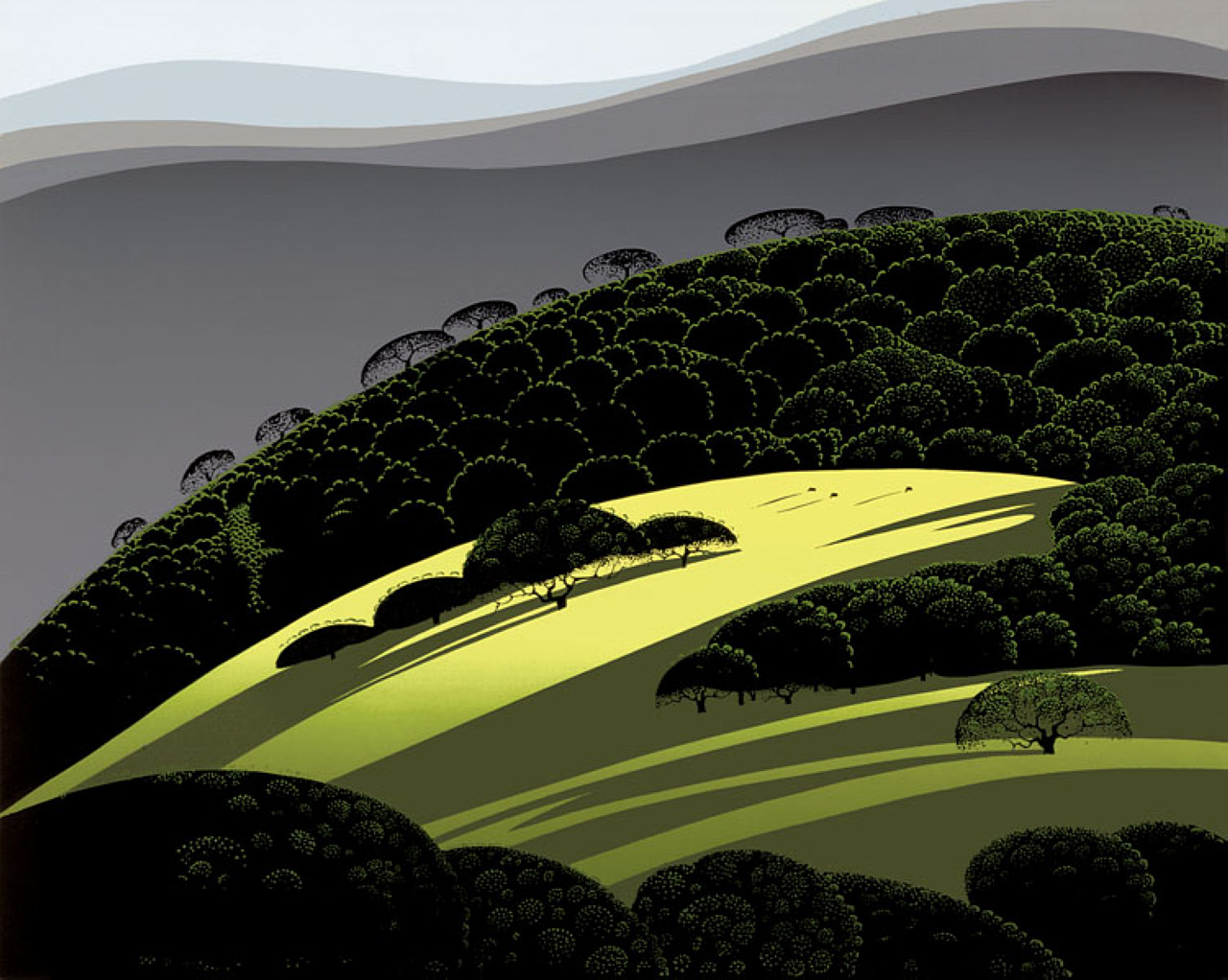The image showcases a serene and beautifully detailed artwork, possibly a painting or a digitally created piece, depicting a lush, light green hillside bathed in sunlight. The open hillside at the center is surrounded by clusters of dark green and black trees, with some positioned in the foreground and others extending into the background, climbing towards the higher parts of the image. The sky above features layered, overlapping clouds in shades of gray and light blue, adding depth to the composition. The background also hints at distant mountains or rolling clouds, enhancing the enchanting, almost otherworldly feel of the scene. The vibrant green grass contrasts sharply with the darker tree tones and the gray sky, making the greenery pop and giving the entire image a peaceful, cartoonish yet realistic quality. This idyllic depiction, free of people and animals, focuses solely on the natural beauty of a sunlit, wooded hillside.